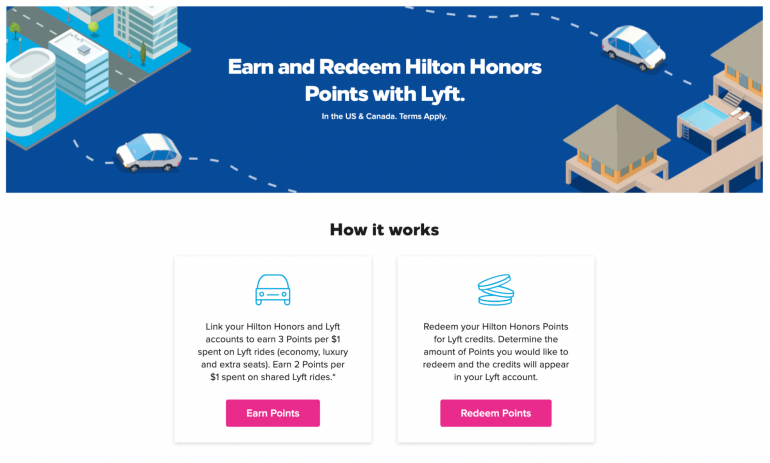This screenshot features a detailed advertisement for a promotional collaboration between Hilton Honors and Lyft. 

At the top, there's a visually engaging banner styled as an infographic depicting a cityscape with various buildings and two cars positioned on the top left and right. Centrally in the banner, bold text states, "Earn and redeem Hilton Honors points with Lyft," with smaller white text below adding, "In the United States and Canada, terms apply."

Beneath this banner, the website background transitions to white. In the middle, in prominent black text, it says "How It Works."

On the left side of the page, there is a white box bordered in gray, featuring a car icon at the top. The text within this box reads: "Link your Hilton Honors and Lyft accounts to earn 3 points per $1 spent on Lyft rides. Economy, luxury, and extra seats earn 2 points per $1 spent on shared Lyft rides." This text is followed by an asterisk, indicating additional terms. At the bottom of this box, there is a pink "Earn Points" button.

To the right, another gray-bordered white box contains an icon of three stacked coins. The accompanying text reads: "Redeem your Hilton Honors points for Lyft credits. Determine the amount of points you would like to redeem and the credits will appear in your Lyft account." This box also features a pink "Redeem Points" button at the bottom.

The overall design is clean and easy to navigate, with each box clearly outlined in gray, emphasizing the distinct sections and functionalities of the promotion.